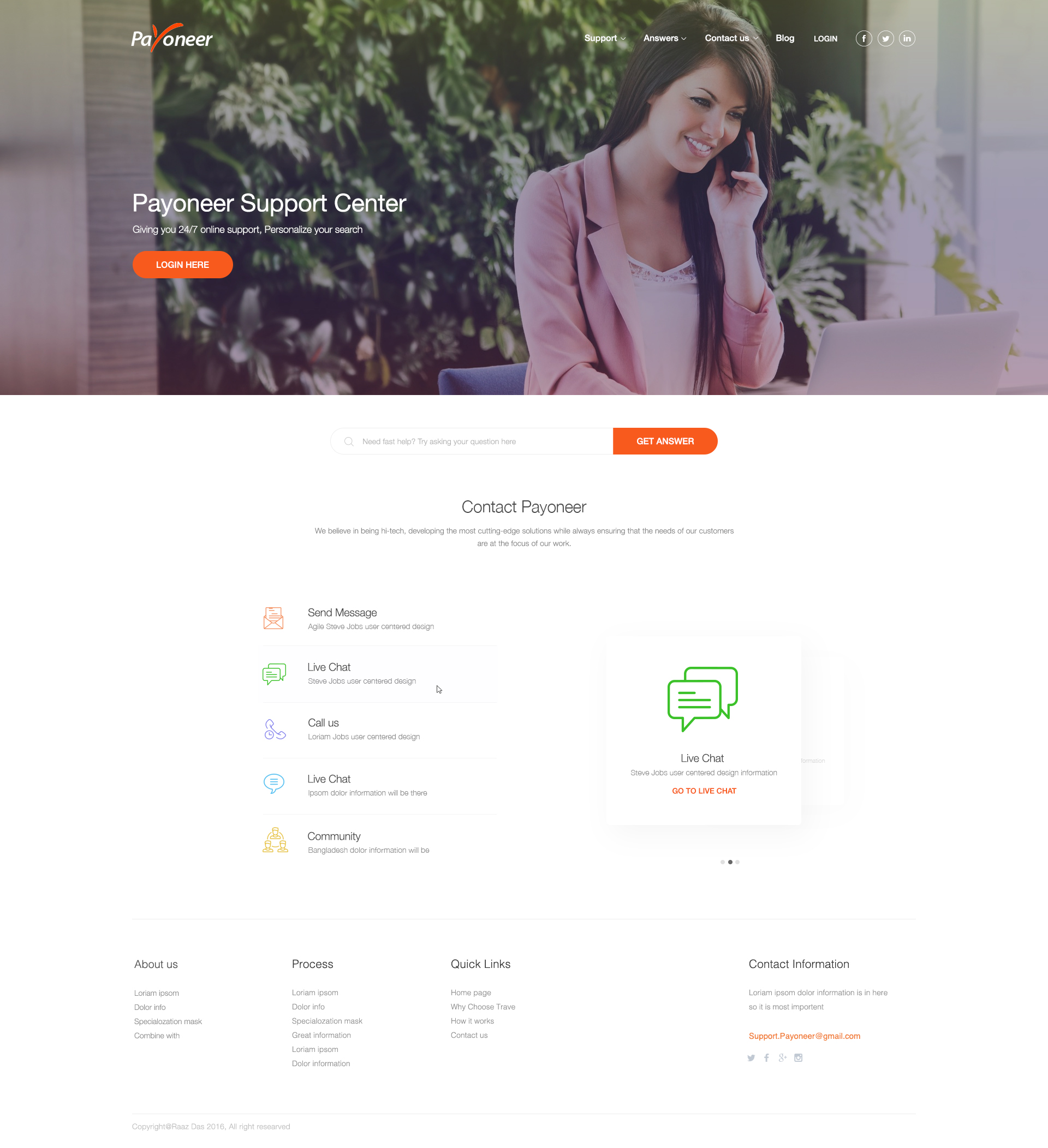The screenshot captures a section of the Payoneer website, prominently featuring their Support Center page. The header at the top showcases a large, slightly blurry image of a woman speaking on her cell phone, spanning the entire width of the page. On the top left corner of this header, the Payoneer logo is clearly visible. Just below, on the bottom left, the words "Payoneer Support Center" are displayed, accompanied by an orange "Join" button directly beneath it.

Transitioning to the main content, the body of the page is predominantly white, providing a clean and uncluttered appearance. Centered immediately below the header image sits a search bar for user convenience. Following this, also centered, is the text "Contact Payoneer."

Further down towards the center-left of the page, there is a horizontal array of contact options, including "Direct Message," "Live Chat," "Call Us," "Live Chat" again, "Community," and "Text Chat." On the right side, a large white box captures attention with a green chat bubbles icon and the label "Live Chat" underneath, indicating an available option for real-time conversation with Payoneer support.